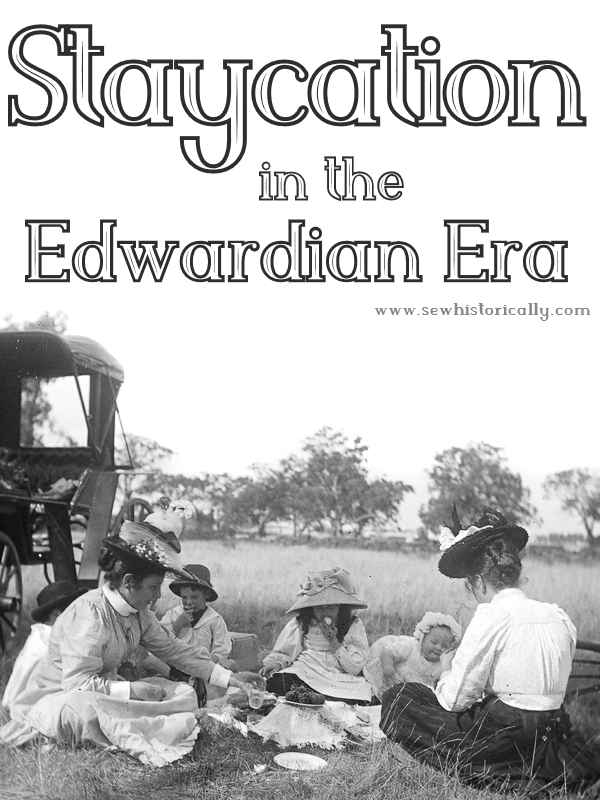In a serene black and white photograph reminiscent of the early 1900s, the scene is set for a "Staycation in the Edwardian Era." At the top of the image, a vintage block print spells out the title, with a reference to www.sewhistorically.com just below it. The focal point of the image features two women and four young children, all dressed in authentic Edwardian clothing. The women are adorned in bonnets while the boys sport regular hats. They are enjoying a leisurely picnic seated on a grassy expanse, with faint, blurred trees providing a natural backdrop. To the left, an open-spoked wheel of a nearby stagecoach hints at their mode of transport, adding to the timeless charm of this idyllic outdoor gathering.